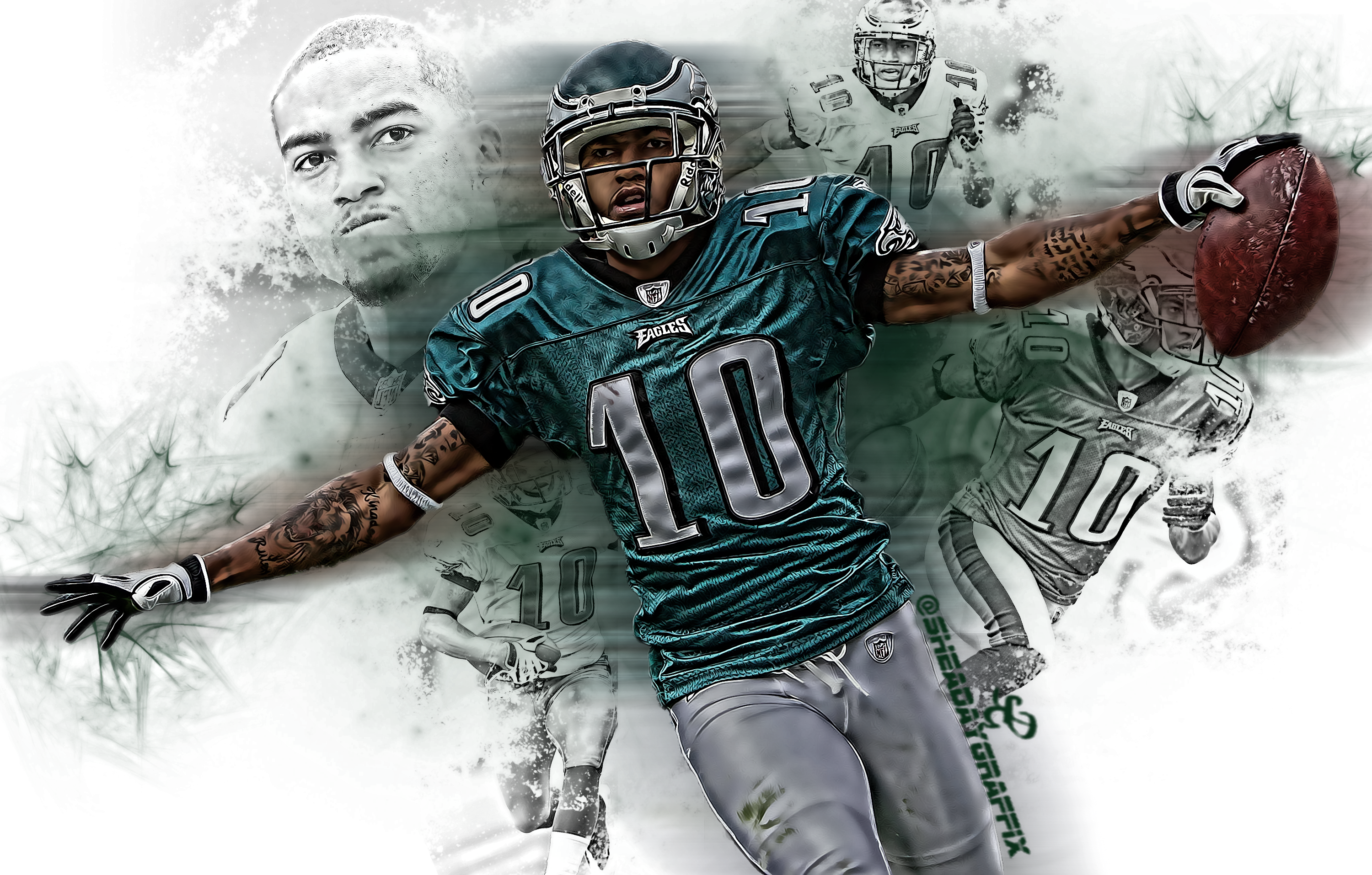The image is a wide rectangular, digitally manipulated photograph featuring a dynamic portrayal of a football player at the center. The main subject, dressed in a metallic dark green jersey with a bold silver '10' and silver pants, appears to be in motion with his body tilted diagonally to the left. His arms are extended outward, mimicking the spread of wings, with his left hand holding a reddish-brown football. He is adorned with black and white gloves, white wristbands around his elbows, and a white and green helmet with additional '10' markings on the shoulders and an eagle design on the sides of his jersey.

Surrounding the central figure are multiple black and white sketches and images of himself performing various football actions, creating a sense of movement and intensity. The background is predominantly white, and the name "Shede Graphics" is boldly printed in green font, aligned vertically along his leg. The overall imagery, including the negative filter effect, enhances the dramatic and artistic presentation of the collage.